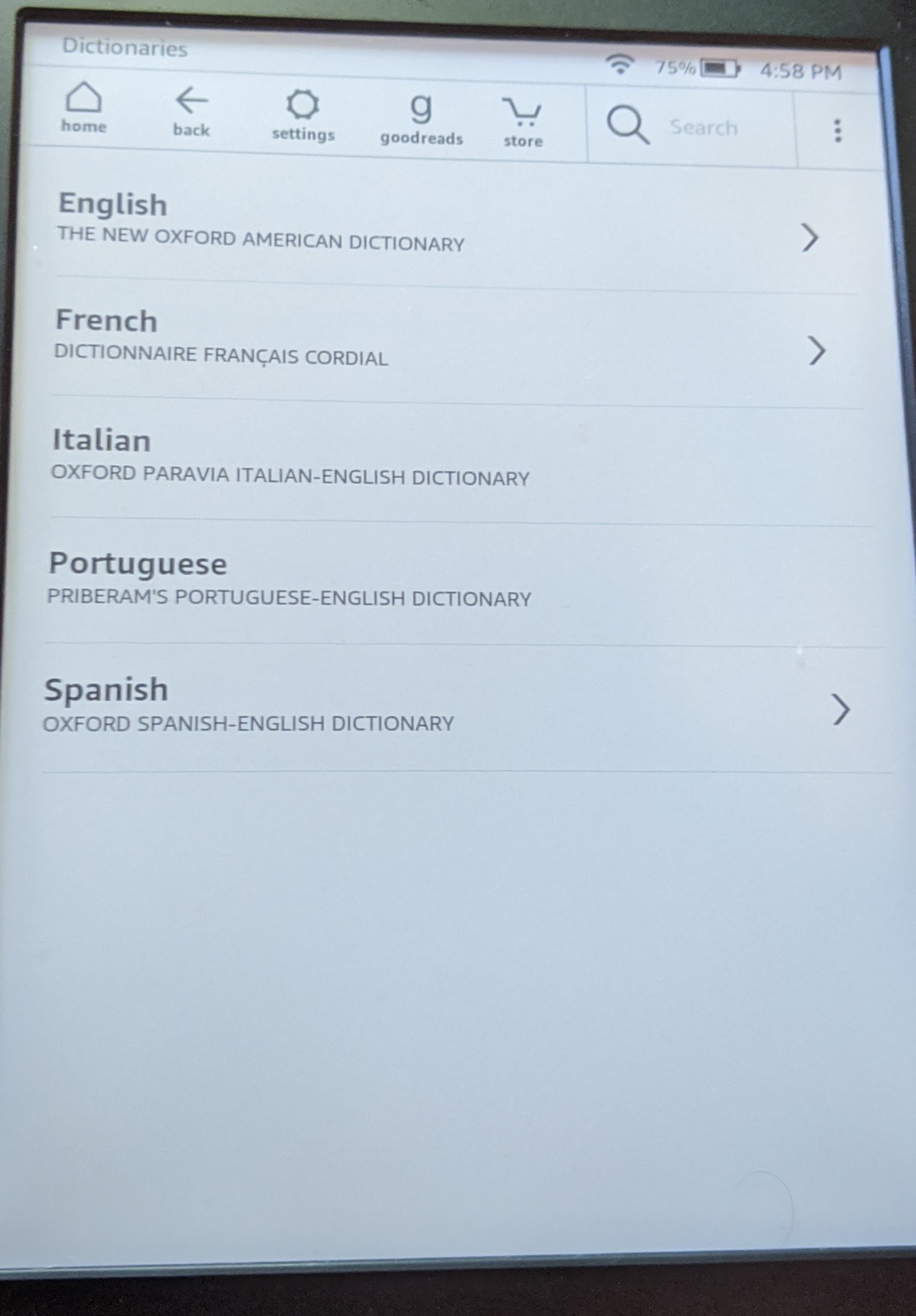In this detailed screenshot of a tablet page, the image is oriented vertically and set against a solid white background. The upper right corner displays the Wi-Fi icon showing a 75% connection, followed by the battery icon, and the time which reads 4:58 p.m. 

On the top left, the word 'Dictionaries' is prominently displayed. Directly beneath it, a navigation bar stretches from left to right, featuring a series of icons and labels: 'Home' accompanied by a home icon, 'Back' with a back arrow above it, a settings icon, 'Goodreads' represented by the letter 'G', and 'Store' with a shopping cart icon. To the right of these, there is a small search box displaying a black magnifying glass icon and the word 'Search' inside it. 

Underneath a light gray line, on the left side in bold black text, the word 'English' is prominently displayed, followed by 'The New Oxford American Dictionary'. Below this, another bold label reads 'French', alongside 'Dictionnaire Français Cordial'.